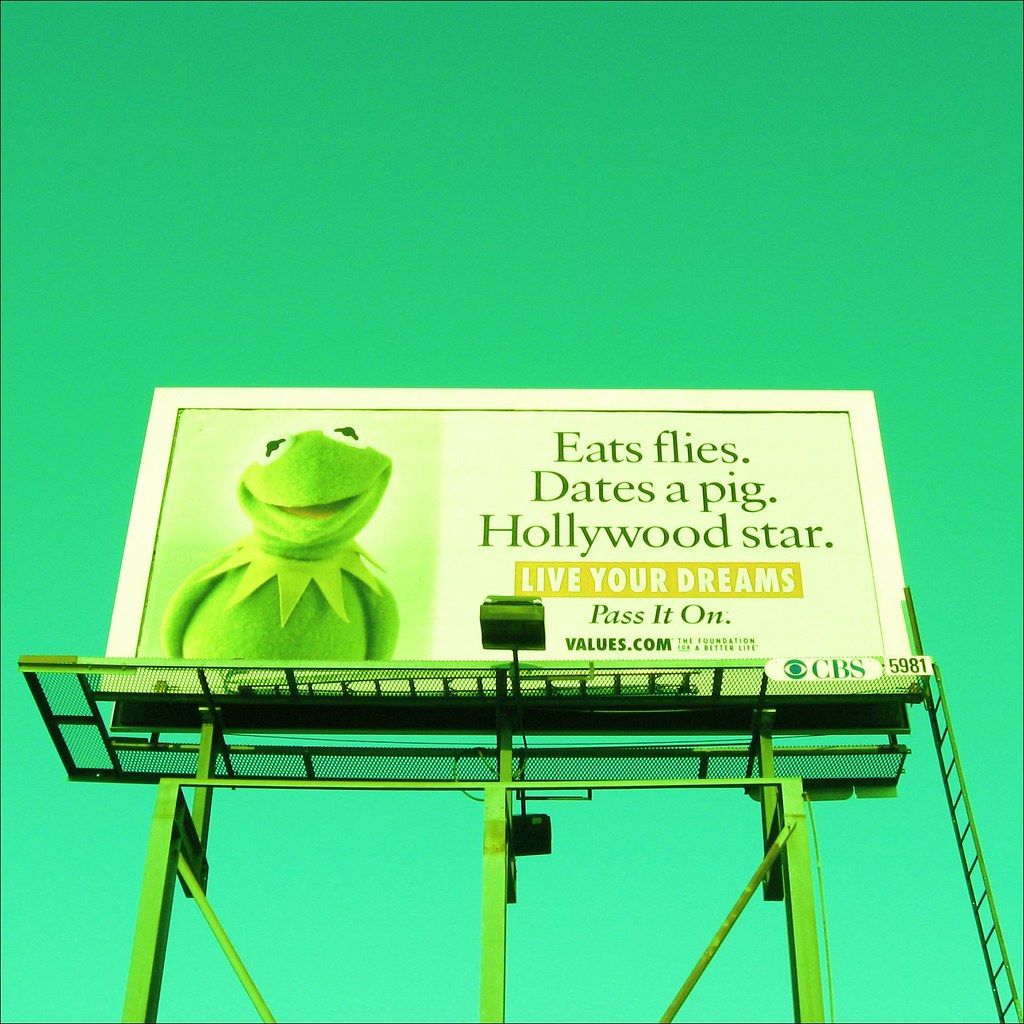The billboard in the image features a bright, chartreuse green background and is elevated on tall stilts with a long ladder leading up to it, suggesting maintenance access. Dominating the left side of the billboard is a smiling Kermit the Frog, easily recognizable by his upside-down triangle collar and his distinctive black-and-white eyes and open red mouth. The billboard has a cream-colored backdrop, accentuated by white edges.

On the right side of the billboard, bold green text reads, "Eats flies. Dates a pig. Hollywood star." Below this, in white lettering set against a mustard-colored strip, the inspirational phrase "Live your dreams" is displayed. Beneath this, in green text, the words "Pass it on" and "Values.com" can be found, along with the mention of "The Foundation for a Better Life." In the lower right corner, the CBS logo along with the network's iconic eye symbol and the number "5981" appear. The billboard is equipped with a light for nighttime visibility, emphasizing its message at all hours.